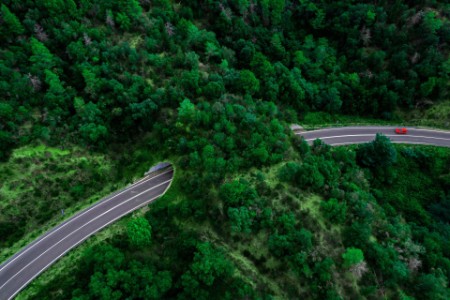This top-down photo, possibly taken from an airplane or helicopter, captures a scenic, curved two-lane road winding through a lush, green landscape. A small red car is visible on the road, though its direction is unclear due to the photo's low resolution. The road is flanked by dense green foliage, suggesting a thriving natural environment. Prominently featured is a nature-formed tunnel or underpass, where trees and bushes arch over the road, creating a verdant canopy. The road markings are distinct, with white lines marking the edges and a double line in the center. The terrain appears steep, particularly around the tunnel area, adding to the picturesque quality of the scene. Despite the image's low resolution, the overall impression is one of rich, varying shades of green interspersed with earthy tones from the visible rocky dirt between the trees.